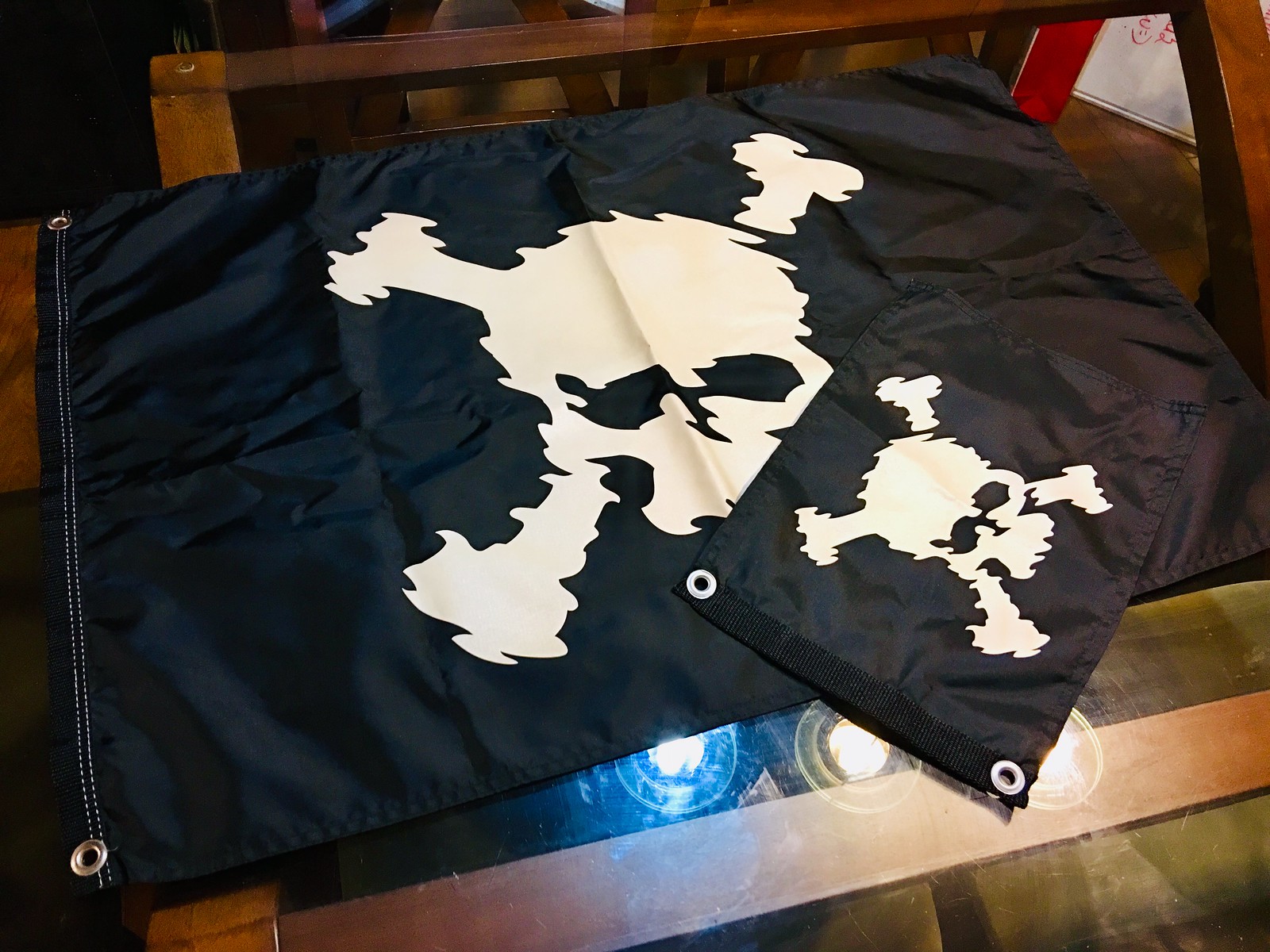This detailed color photograph, taken from above, showcases two black vinyl flags featuring a stylized white Jolly Roger Skull and Crossbones logo. The flags are laid out on a glass-top coffee table with a wooden frame, visible along the perimeter. The larger flag, at the bottom, shows creases from storage and has metal rivets at the top left and bottom right corners for mounting. Its Skull and Crossbones design appears wavy and smeared, adding a unique, distorted effect. On top of this flag lies a much smaller version, approximately a fourth of the size, also with metal rivets and the same white stitched design, featuring the wavy outline around the skull and crossbones. Reflections from three overhead spotlights—blue and yellow—can be seen on the glass surface beneath the flags. The scene gives a clear view of the wooden frame of the table, adding a rustic touch to the modern pirate-themed flags displayed.